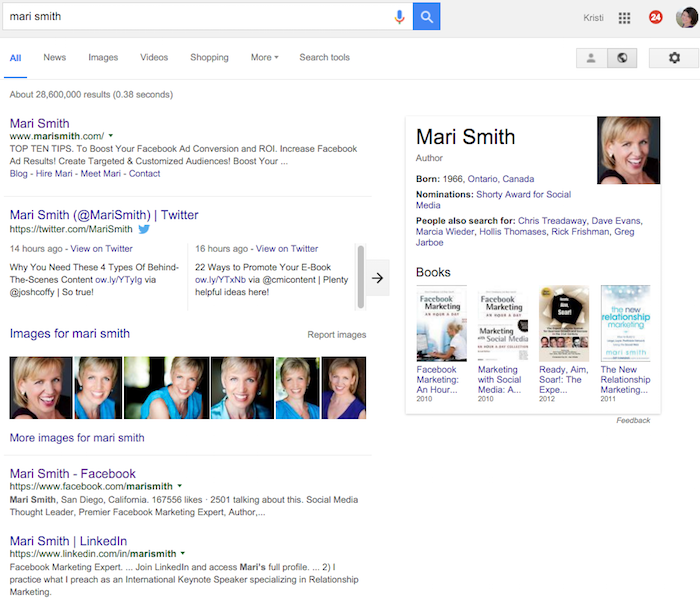This detailed image depicts a search results page for 'Mary Smith' on a website. At the upper left-hand corner, a rectangular search box displays the query 'Mary Smith.' Adjacent to it, a microphone icon is situated on the right. Next to the microphone, there is a blue search button featuring a magnifying glass icon. On the far right of this section, the name 'Christie' is displayed, beside which lies a grid icon composed of nine smaller squares. Further right, there's a red circle reading '24,' and beside it, a profile picture of a brunette woman, appearing to be a white female.

Below this, a series of tabs are underscored, including 'All,' 'News,' 'Images,' 'Videos,' 'Shopping,' and 'More' with a drop-down arrow. To the right of these tabs, three icons are visible. The search results mention approximately 28,600,000 results beneath these tabs.

The primary highlighted result features the name 'Mary Smith' along with the URL 'www.MarySmith.com,' which includes a drop-down arrow and related content. Following this, there is a link to Mary Smith's Twitter account, displaying the handle '@MarySmith' and a note that it was updated '14 hours ago.'

Further down, a section labeled 'Images for Mary Smith' exhibits six images. Additional links include 'Mary Smith Facebook' and 'Mary Smith LinkedIn,' each accompanied by relevant information.

On the right-hand side, an information panel highlights 'Mary Smith' as an author, with a photograph of her, as well as details about her age and books.